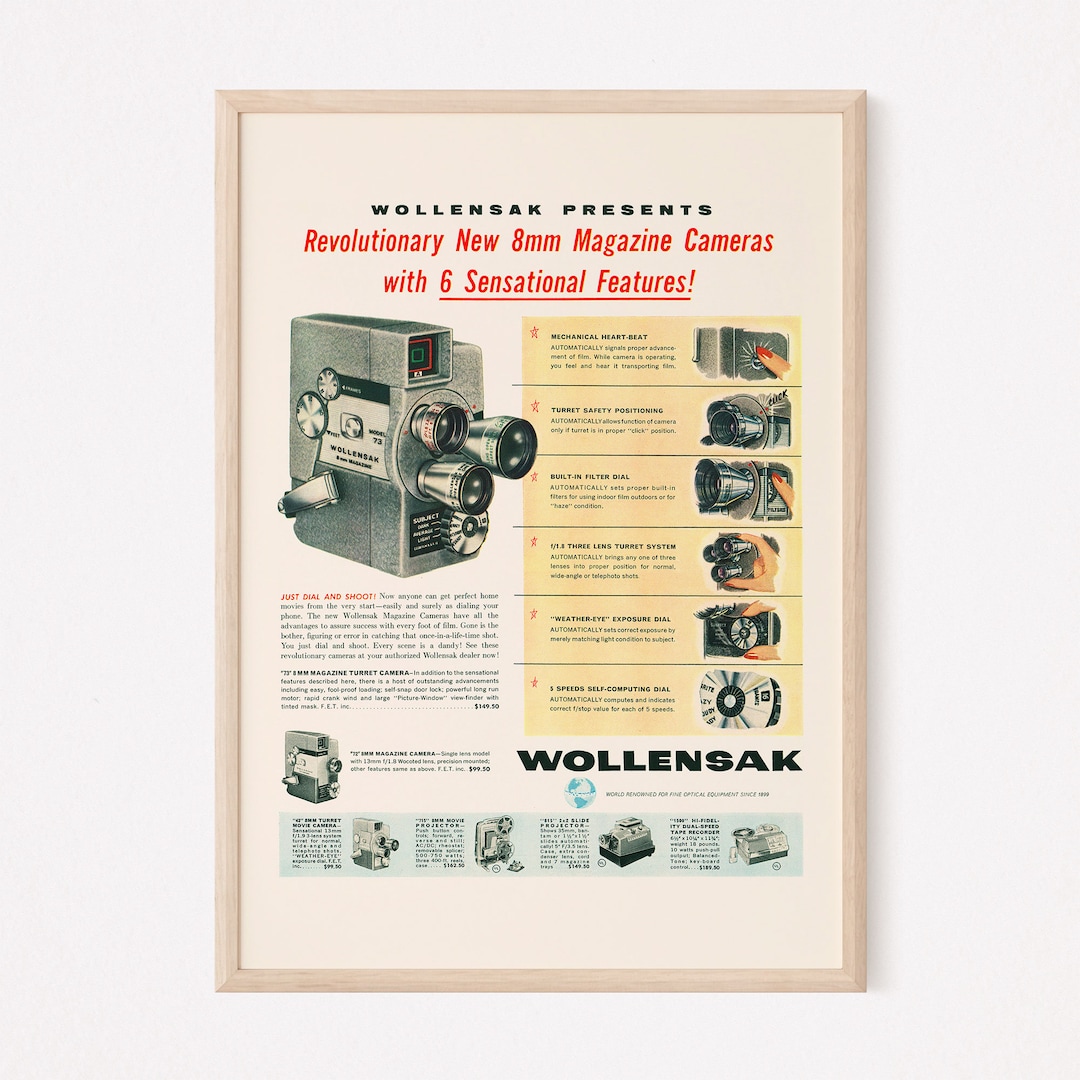The image shows a well-lit, framed advertisement mounted on a white wall. The frame appears to be a light wooden color. The central text in black and red reads: "Wallensack presents revolutionary new 8mm magazine cameras with six sensational features." On the left side of the image, an old-fashioned camera with a three-lens turret system is prominently displayed. The right side features smaller images and text detailing the camera's features, which include a mechanical heartbeat, turret safety positioning, built-in filter dial, weather eye exposure dial, and five-speed self-computing dial. Below the camera, there's a paragraph describing it as a "8mm magazine turret camera," priced at $149.50, reflecting the advanced and expensive nature of the device at the time. Despite the detailed presentation, some of the text is small and difficult to read, affecting the clarity of the advertisement's finer points.